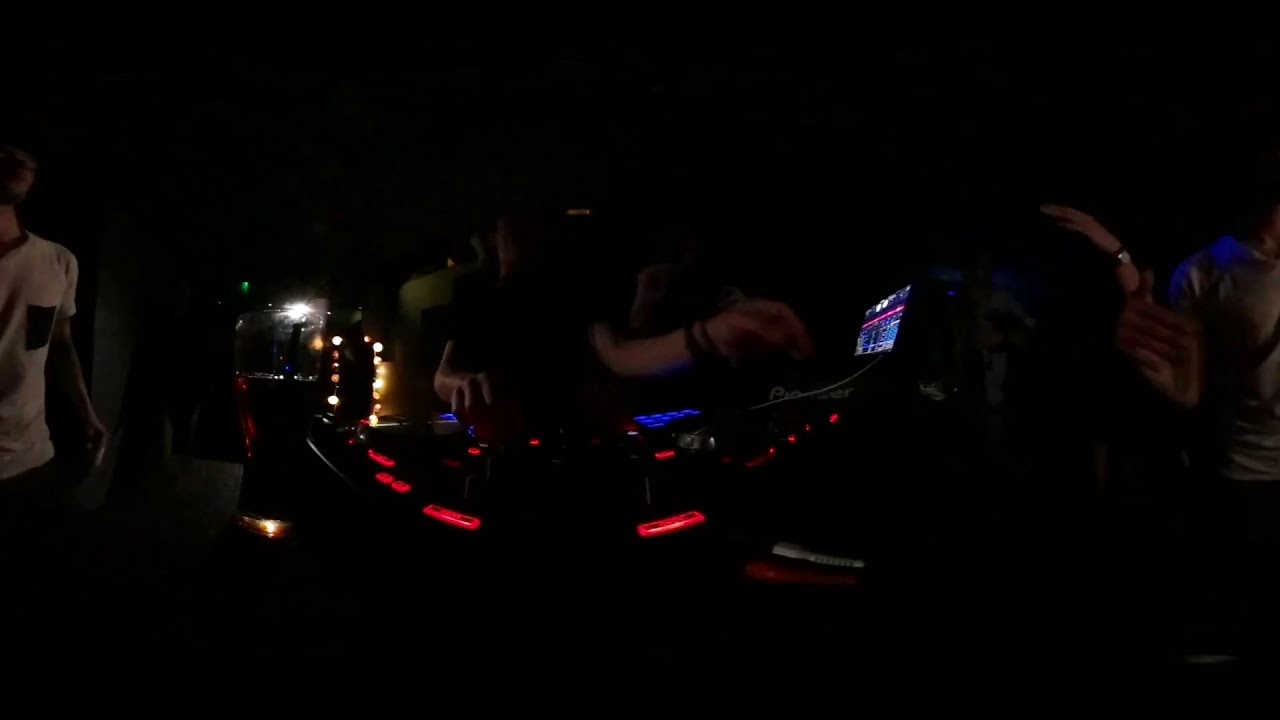The photograph captures a dark nightclub setting where a DJ is performing. The dimly lit room makes it challenging to discern details, but the scene features the DJ standing at a soundboard illuminated by red and blue lights. The DJ is wearing a black short-sleeved t-shirt and bracelets on their left wrist, though their face remains indistinguishable. In the background, a white light on the wall, possibly an emergency exit light, casts a faint glow. On the left side, a person in a white t-shirt with a black chest pocket seems to be moving, perhaps heading back to the dance floor. From the right side of the image, the raised hands of dancing club-goers are visible. The 360-degree perspective adds to the distorted, dynamic view of the DJ's setup, emphasizing the vibrant yet subdued nightlife atmosphere.